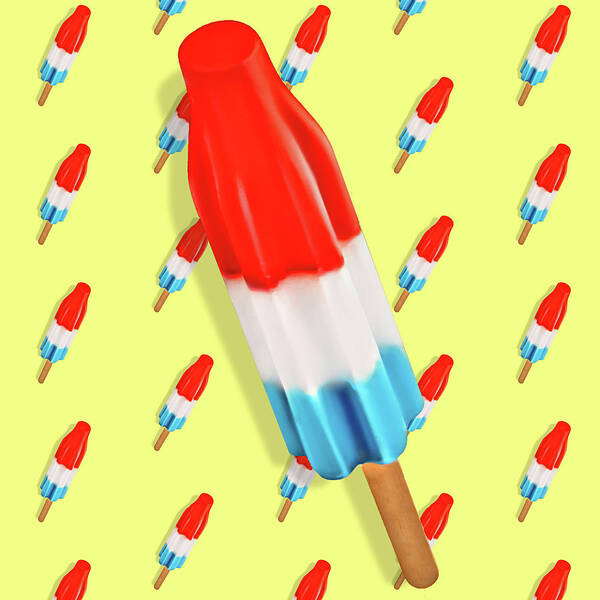The stylized, cartoonish image resembles a photorealistic painting at first glance. It depicts a vibrant display of red, white, and blue popsicles, commonly known as Rocket Pops. The centerpiece is a large popsicle angled slightly to the left, reminiscent of a rocket ascending into the sky. Encircling this prominent popsicle, the background features multiple smaller, identical popsicles, arranged in about five diagonal rows slanting 45 degrees to the right. The popsicles are set against a pale yellow backdrop, highlighting their vivid colors and evoking a sense of summer nostalgia. The blue section is at the bottom, white in the middle, and red at the top, echoing the classic flavors of berry, lemon or pineapple, and strawberry, respectively.